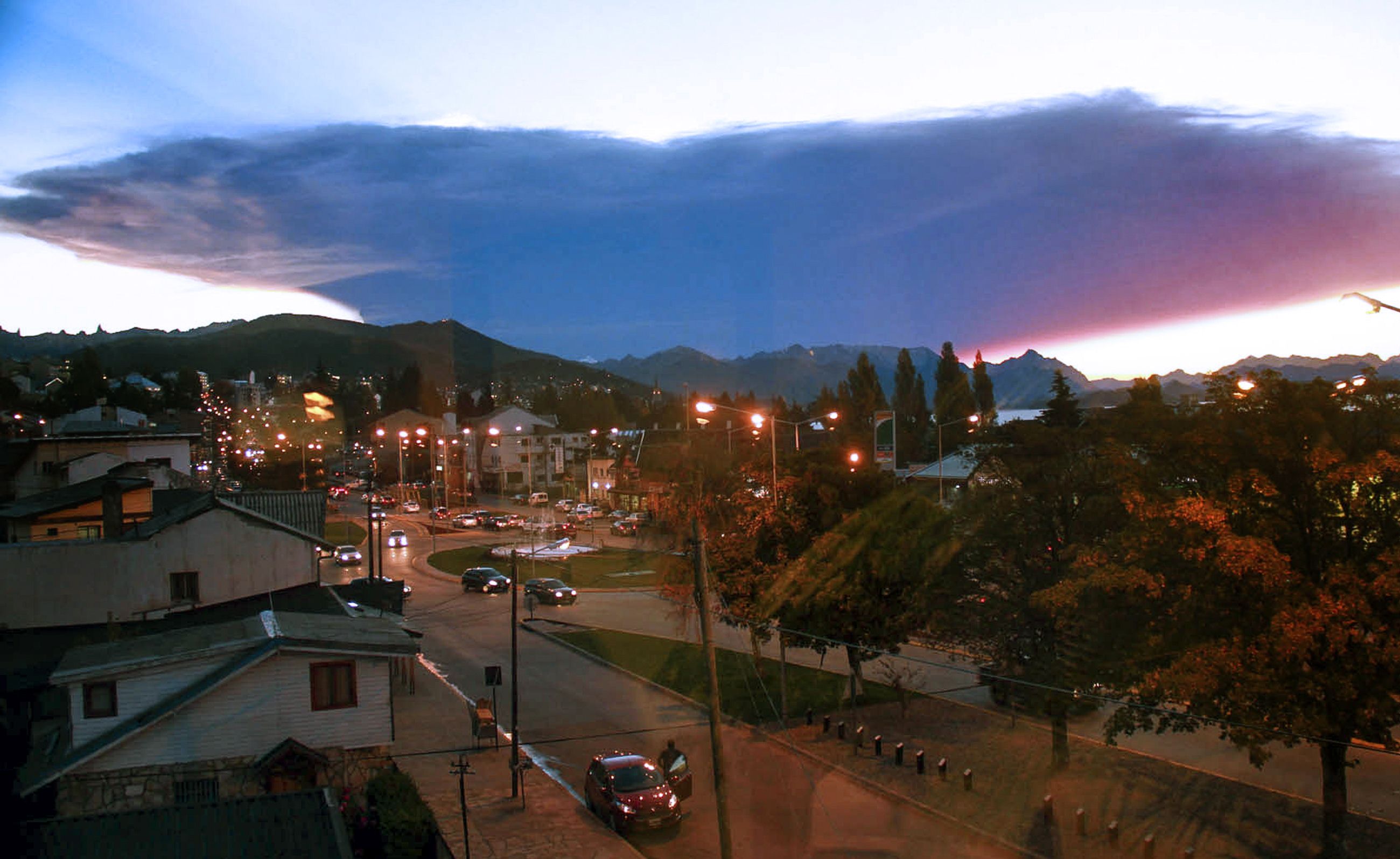This image presents a stunning nighttime aerial view of a medium-sized town. The scene is dominated by a vast, dark gray cloud arching across the sky, casting shadows over the rolling hills and mountainous range in the distance. The clear blue sky with scattered thin white clouds adds a contrast to the darker cloud below.

The town itself is bustling with activity, illuminated by numerous city lights. The main road, busy with cars, is a focal point, with a distinctive red car in the center where a man is getting out. This main thoroughfare is lined with trees and patches of grass, and there is a visible side street forming a V shape, surrounding a grassy area bordered by concrete curbs. Streetlights and house lights are turned on, indicating it is either dusk or dawn.

On the left side of the main street, numerous houses with white siding and green roofs are visible, extending into the distance and giving the impression of a quaint, little town. The town appears to be nestled amongst green trees and has a serene lake visible far off. Road signs and additional cars navigating the circular roadway add to the complexity and realistic feel of the townscape.